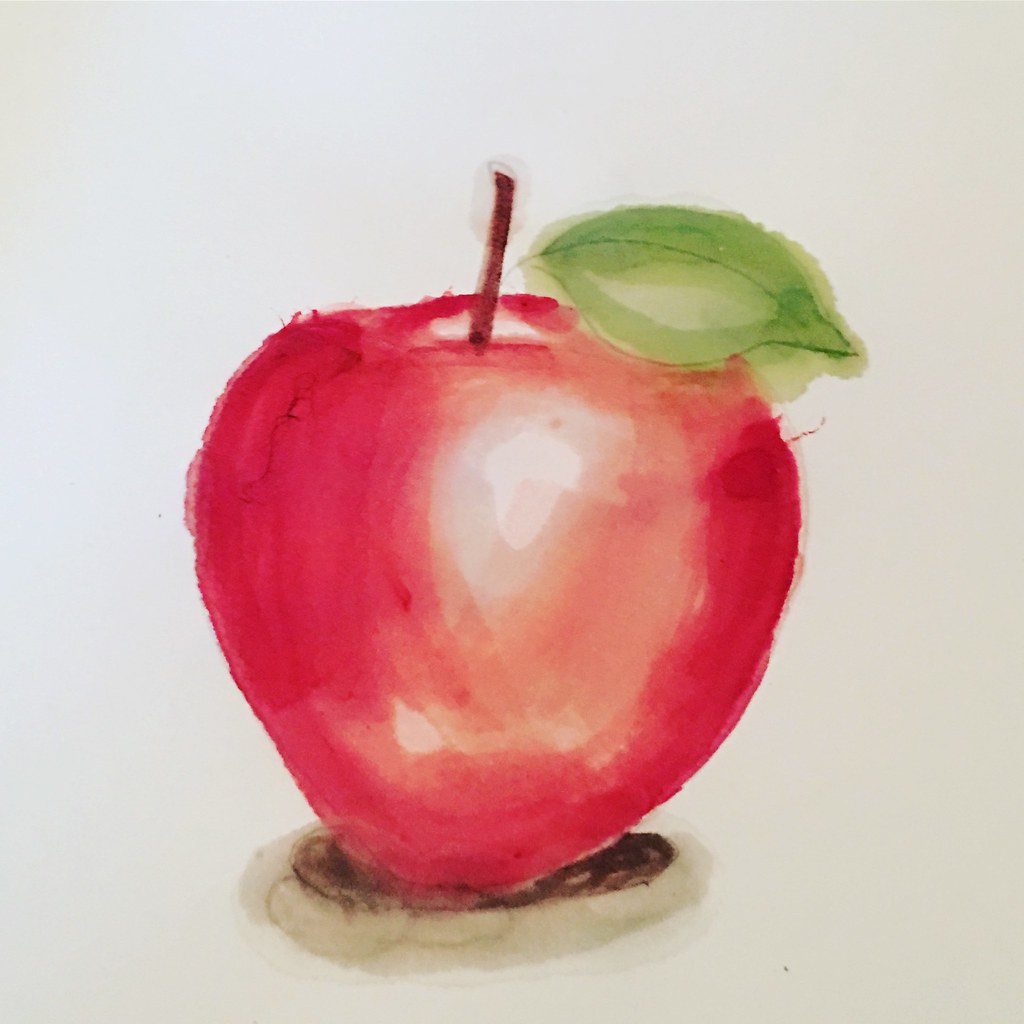This image is a slightly taller-than-wide, square-like painting of a vibrant red apple. The apple features a prominent shiny spot near the center, slightly off to the right, contributing to its lifelike appearance. At the top of the apple, a brown stem extends upwards, culminating in a green leaf that stretches from the left to the right, occupying the upper right section of the fruit. The apple rests on a disk resembling the top of a toasted English muffin. The painting, likely created using either acrylics or watercolors, exhibits a slightly blotchy texture that enhances its realistic yet artistic charm. The green stem, in particular, shows the delicate nuances of watercolor technique. The background is a stark, clean white, making the colorful details of the apple stand out.